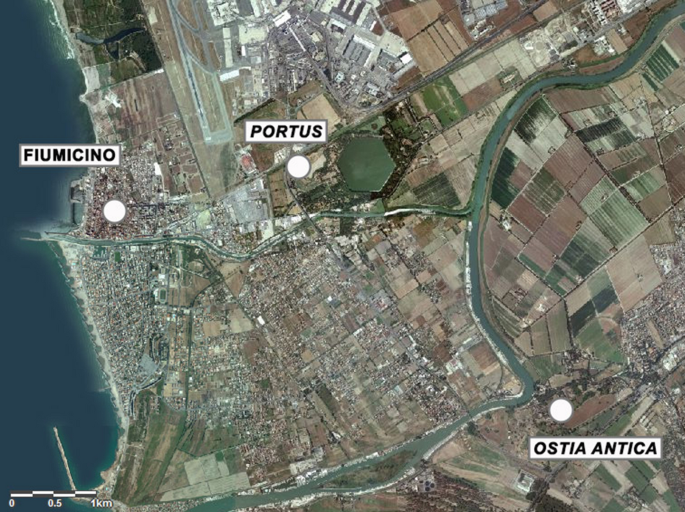This highly detailed aerial photograph, resembling a Google Maps screenshot, showcases a coastal region, likely captured from an airplane or helicopter. On the left side of the image, there is a vast blue expanse of water, which could be an ocean or a lake. A river can be seen cutting through the landscape, flowing towards the water body. The land is divided into various fields and sections of arable land, with the tops of houses, grassy areas, and dirt patches visible. Three distinct white markers label different cities: Fiumicino, located near the coast on the left, Portus in the middle of the image, and Ostia Antica at the bottom right. The scale at the bottom of the image indicates distances ranging from 0 to 1 kilometer.